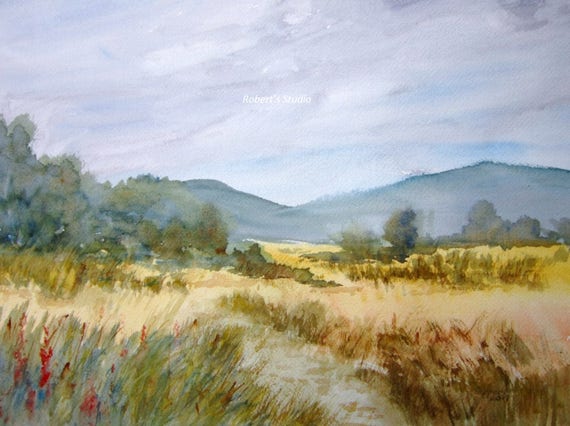This horizontal watercolor painting depicts a serene pastoral landscape with nuanced detail. In the foreground, long grasses, predominantly in hues of yellow, tan, and muted greens, gently sway, punctuated by small patches of red and blue flowers near the bottom left corner. Transitioning to the middle ground, clusters of trees and shrubs provide a verdant, textured layer of greenery that contrasts with the simplicity of the grasslands. In the distance, the soft silhouette of hills, possibly barren mountains, adds depth to the scene. The sky above is predominantly gray and cloudy, with subtle hints of blue, merging seamlessly with the white in the clouds. Despite its muted color palette, featuring browns, tans, greens, and light touches of white and blue, the painting is rendered with considerable skill. A barely discernible watermark in the sky appears to read "Roberts Studio."